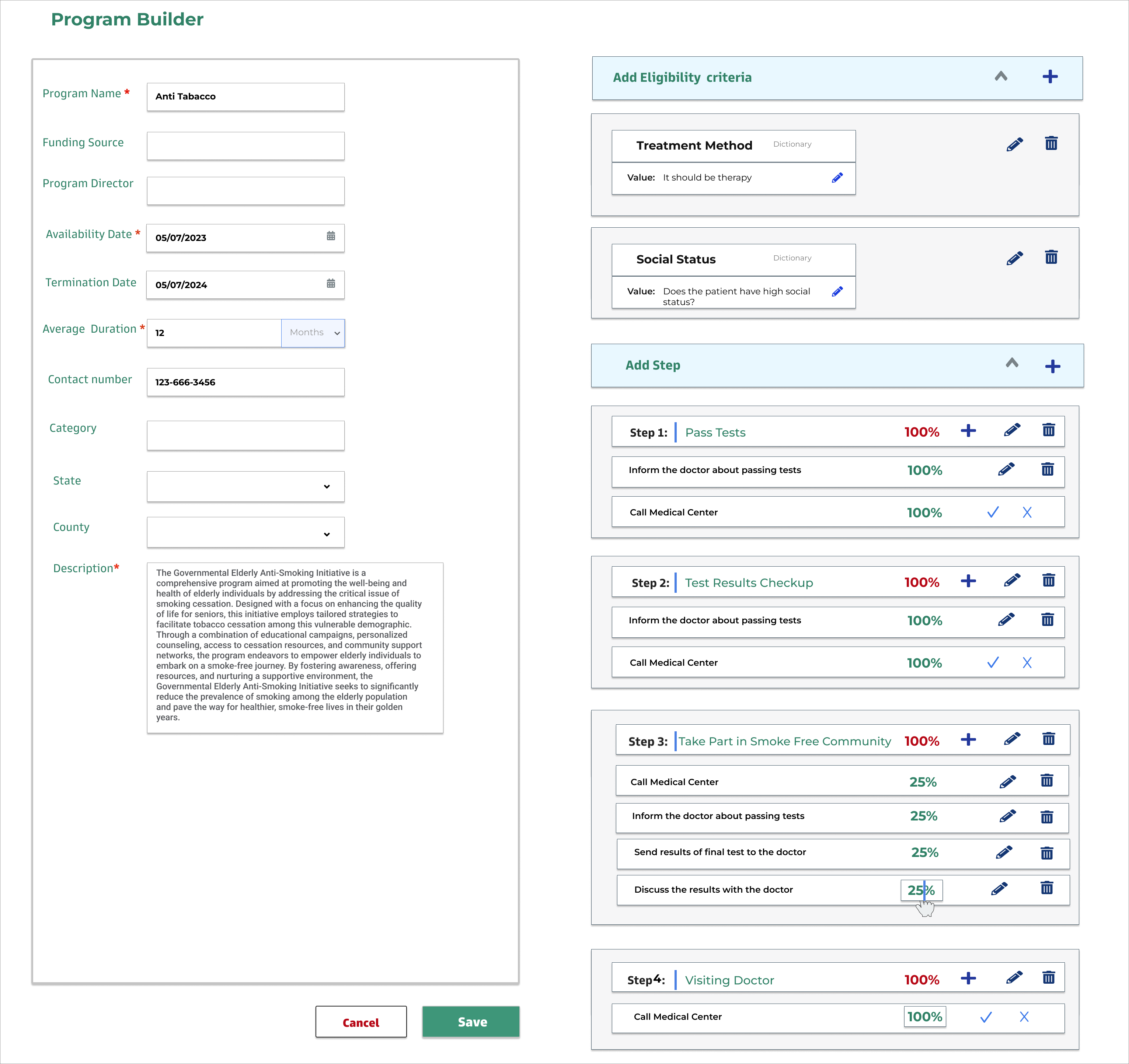The image displays a comprehensive program builder interface with a gray border. The upper left corner features the label "Program Builder" in gray. Inside a darker gray box, there are various fields: 

1. **Program Name:** Listed as "Antsy Tobacco" in black text.
2. **Fundraising Source:** Not specified.
3. **Director:** Not specified.
4. **Available Date:** 05/07/2023.
5. **Termination Date:** 05/07/2024.
6. **Average Duration:** 12 months.
7. **Contact Number:** 123-666-3456.
8. **Category, State, County:** Not specified.
9. **Description:** Contains an overwhelming amount of text that is illegible.

At the bottom right, there are two buttons: 
- **Cancel:** Black text on a white background.
- **Save:** Teal text on a white background.

On the right-hand side, there is a section dedicated to the "LV Treatment Method" with a focus on social status. This section contains steps divided as follows:
- **Step 1:** Consists of one item.
- **Step 2:** Consists of one item.
- **Step 3:** Consists of four items.
- **Step 4:** Consists of one final item.

Each step includes various tasks that collectively sum up to 100%. 

The interface is densely packed with information, making navigation potentially overwhelming.